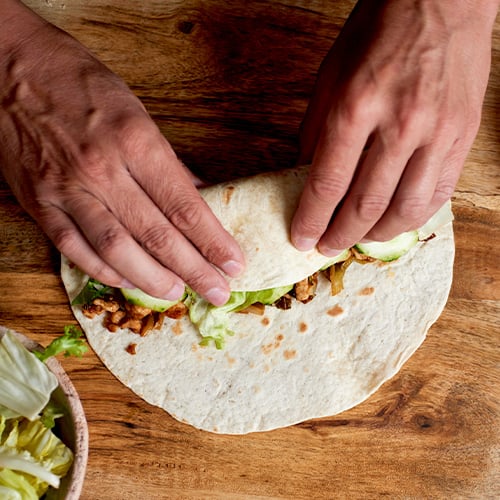This close-up photograph captures the hands of a person, likely a Caucasian man, in the process of folding a burrito on a rustic, lightly varnished wooden table with a prominent grain pattern. The man's hands are engaged in tucking and rolling the burrito away from him, showcasing deft culinary skills. The burrito, wrapped in a homemade-looking flour tortilla, contains visible ingredients such as cucumber slices, lettuce, meat, and possibly beans. To the left of the burrito, we see a small wooden bowl partially in the frame, containing cut-up iceberg lettuce. The image focuses on the nearly finished burrito and the hands up to the wrists, providing a detailed view of this meal preparation scene.